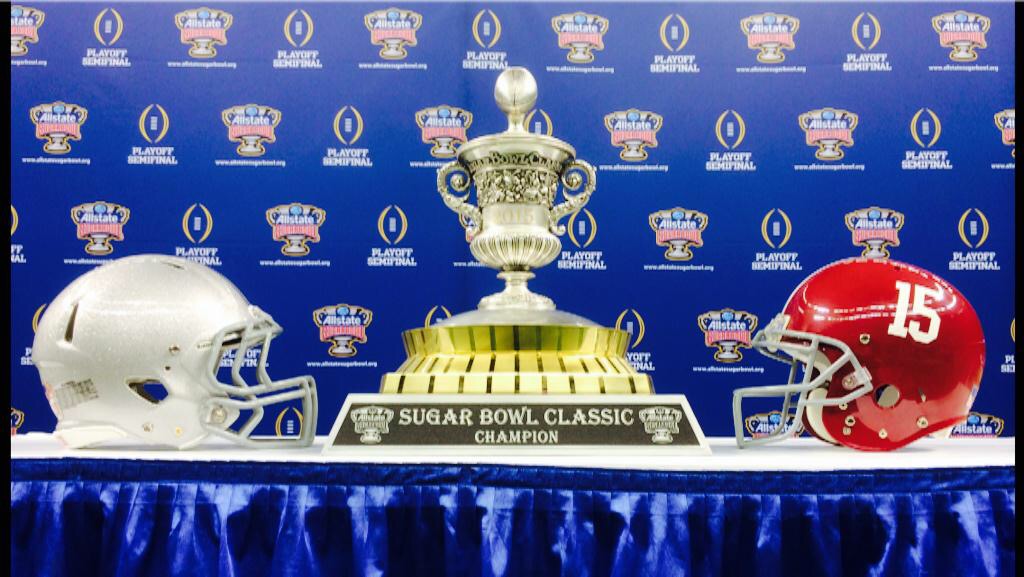The image depicts a press conference setup for the Sugar Bowl Classic Championship, akin to the Super Bowl but for the distinguished Sugar Bowl event in American football. Centered on a small white table draped in gathered blue satin fabric, there is a large, ornate, silver urn-shaped trophy with two prominent handles and a flared base, topped with a grand silver ball. This trophy, designated for the "Sugar Bowl Classic Champion," is the focal point of the display, with a matching plaque situated in front highlighting the trophy’s name. Flanking the trophy are two American football helmets: the left helmet is solid white while the right is bright red featuring the number 15. The backdrop consists of a blue marketing media board adorned with horizontal lines of the "Playoff Semi-Final" text and All-State logos, commonly seen at sporting events to display sponsors.